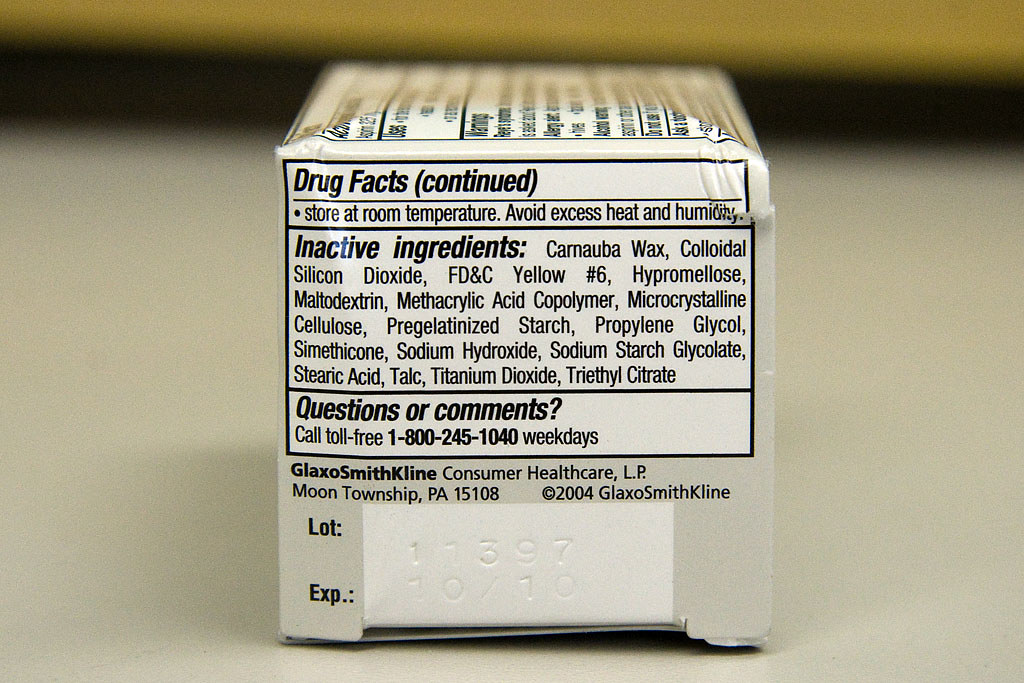The image captures the bottom portion of a box of medication, likely aspirin or similar pills. Displayed prominently are the drug facts and additional product information. The "Drug Facts" section highlights storage instructions, advising to keep the product at room temperature and to avoid excessive heat and humidity.

The list of inactive ingredients includes: carnauba wax, colloidal silicon dioxide, FD&C Yellow No. 6, hypromellose, maltodextrin, methacrylic acid copolymer, microcrystalline cellulose, pregelatinized starch, propylene glycol, simethicone, sodium hydroxide, sodium starch glycolate, stearic acid, talc, titanium dioxide, and triethyl citrate.

For any questions or comments, customers are directed to call the toll-free number 1-800-245-1040 on weekdays. The product is manufactured by GlaxoSmithKline Consumer Healthcare, LP, located in Moon Township, PA 15108, as noted by the copyright 2004 GlaxoSmithKline mark on the box. Additionally, the box is imprinted with the lot number 11398 and indicates an expiration date of October 2010. The entire package is placed on a countertop.